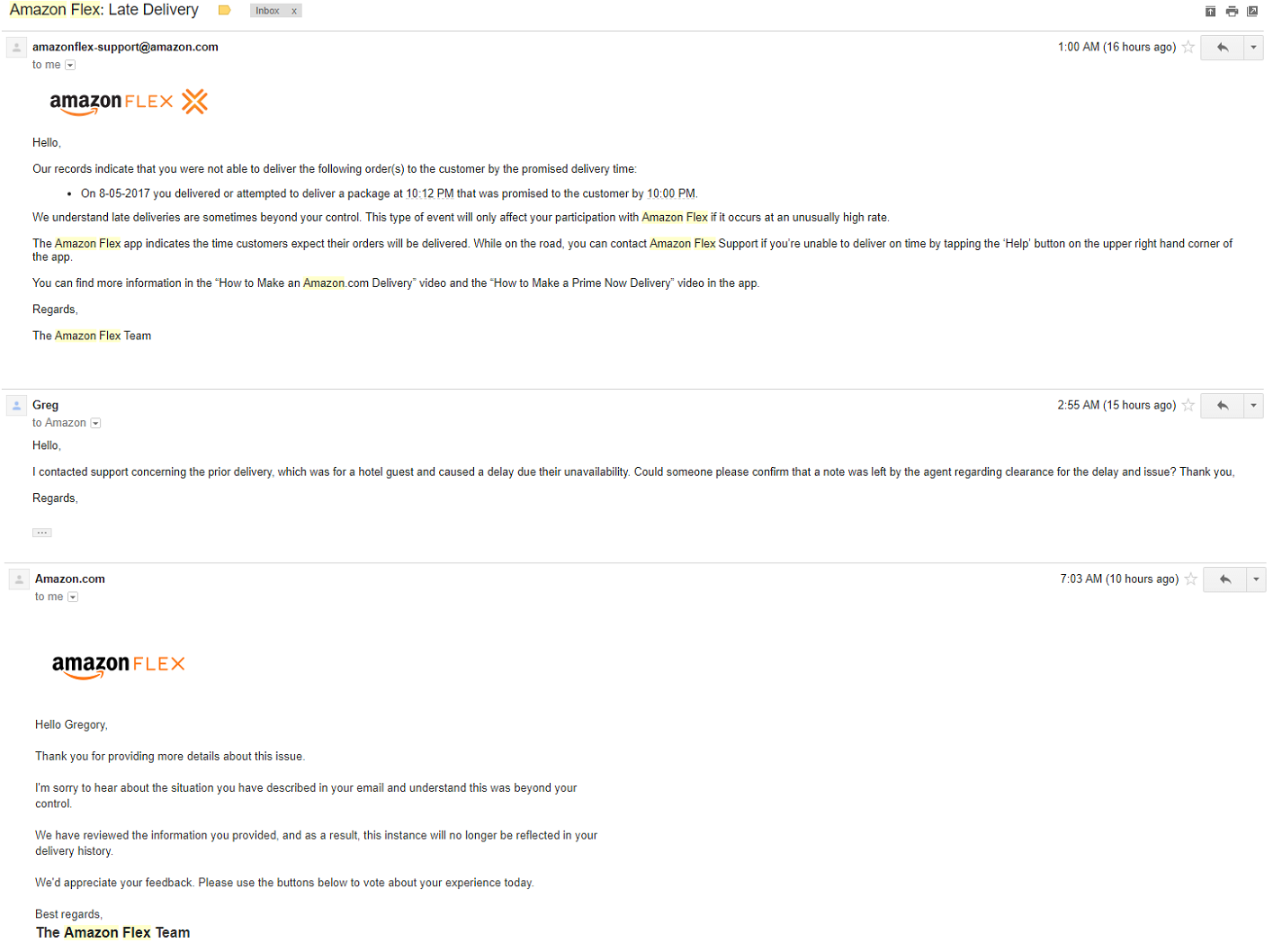This image is a detailed screenshot of an email chain between an individual named Greg and Amazon Flex Support. The email chain is under the subject: "AmazonFlexLateDelivery." It begins with a message from Amazon Flex, stating: 

"Hello, our records indicate that you were not able to deliver the following orders to the customer by the promised delivery time. On August 5, 2017, you delivered or attempted to deliver a package at 10-12 pm that was promised to the customer at 10 pm. We understand that late deliveries are sometimes beyond your control. This type of event will only affect your participation in Amazon Flex if it occurs at an unusually high rate." 

The email continues with advice on how to make timely deliveries and offers links to helpful videos.

Greg then responds: 

"Hello, I contacted support concerning the prior delivery which was for a hotel guest and caused a delay due to their unavailability. I'm pleased to confirm that a note was left by the agent regarding clearance for the delay and issue. Thank you."

Amazon Flex Support follows up with: 

"Thank you for providing more details about the issue. Sorry to hear about the situation you described. We have reviewed the information you provided and as a result, this instance will no longer be reflected in your delivery history."

This email exchange illustrates an individual's experience with Amazon Flex, highlighting the system's responsiveness and human-like consideration in handling specific delivery issues. By reviewing Greg's situation and removing the late delivery mark from his account, Amazon Flex Support shows a level of understanding and flexibility.